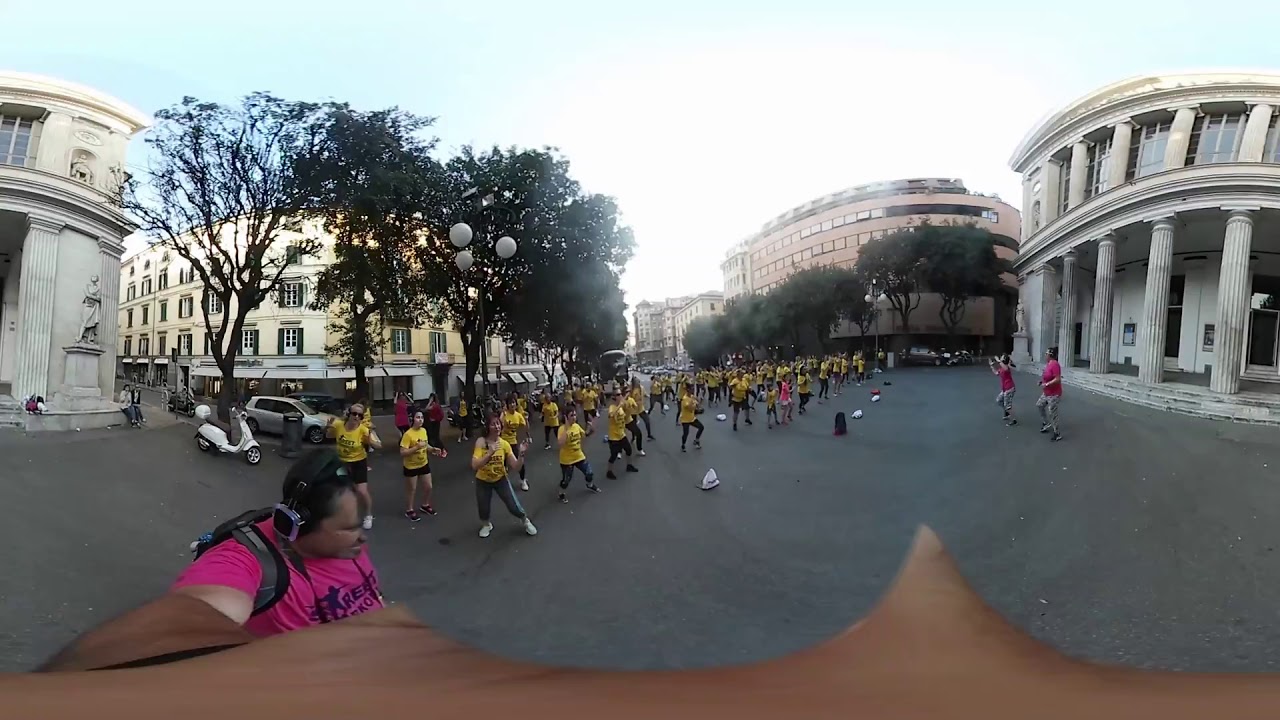The photograph captures a bustling street scene during the daytime, showing a wide paved street flanked by buildings on both sides. On the right-hand side, a prominent white two-story building with large columns dominates the foreground, and further down, a rounded building with trees lining its side can be seen. On the left-hand side, there's the edge of another white building and adjacent to it, a building partially obscured by trees, in front of which some balloons are caught in the branches.

Occupying the street are numerous individuals in yellow t-shirts and black pants or shorts, organized in several rows of three, starting from the foreground and extending into the distance. The individual closest to the camera is slightly turned to the right, while further down the rows, many participants appear to be engaged in a coordinated activity, possibly dancing or exercising. Directing this activity, two individuals in pink t-shirts and khaki or gray pants face the lines of people in yellow.

At the bottom left corner of the image, another person in a pink t-shirt and a backpack with over-the-ear headphones extends their arm towards the camera, creating a slightly distorted effect due to the photography stitching process. This individual's arm appears elongated and wavy. Additionally, there is a brown tarp-like object extending across the bottom of the image from left to right. The entire scene is set against a backdrop of a very light blue sky, with a bright white half-sphere suggesting the presence of the sun.